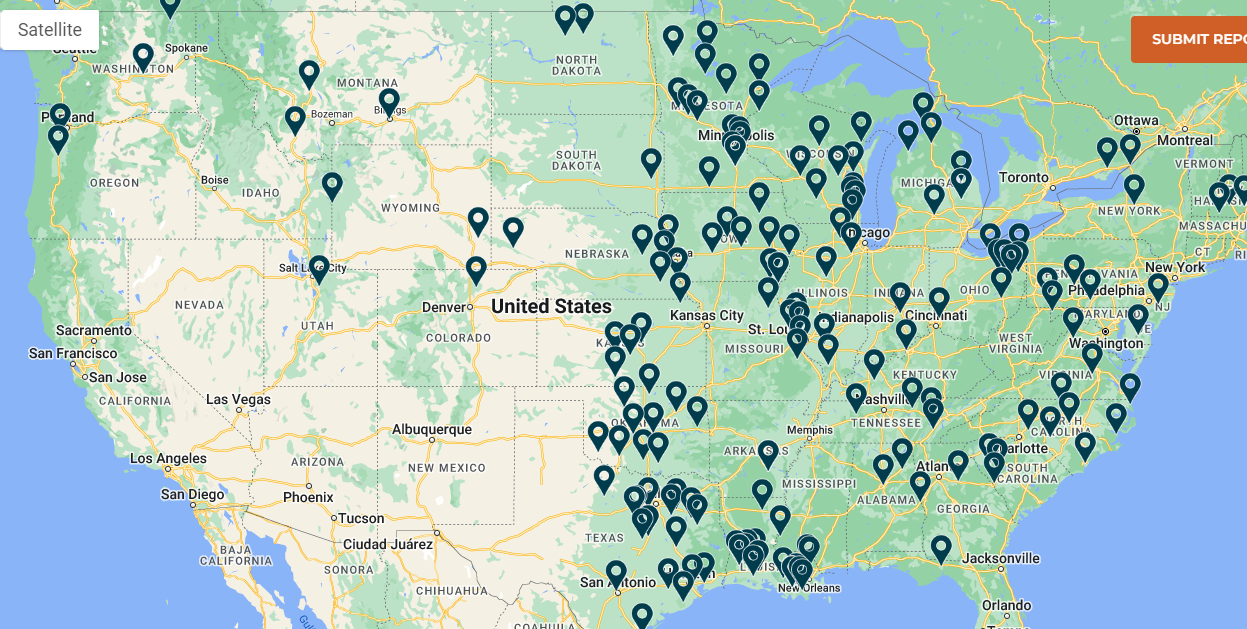This image is a detailed satellite map of the United States with a blue background. Prominently, it features an assortment of colors to depict various landscapes: green areas signify grassy regions, while lighter, beige hues represent desert regions. Notable elements on the map include a white rectangle labeled "Satellite" in the upper left-hand corner and an orange rectangle labeled "Submit Report" in the upper right-hand corner. The right-hand side of the map is dotted with numerous blue teardrop-shaped pins, suggesting locations that have been searched or marked for a specific purpose. These markings are sparse in states like Oregon, Washington, Idaho, Montana, Utah, Colorado, Nebraska, and Wyoming, but they become denser from the Midwest to the East Coast, indicating a higher concentration of interest or activity. Additionally, this map extends beyond the U.S. borders to include parts of Canada, with cities such as Montreal, Ottawa, and Toronto labeled. In the U.S., notable Californian cities and state capitals like those of Nevada, New Mexico, and Arizona are also identified. Yellow routes demarcate major freeways crisscrossing the map, further enhancing the detail and utility of this comprehensive geographic representation.